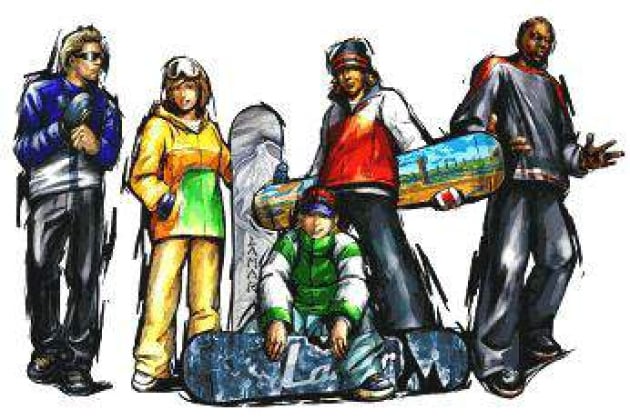The image depicts a stylized, digital drawing of five cartoon snowboarders on a white background, exuding a retro vibe reminiscent of the 70s or early 80s. The group, appearing to be in their late teens or early 20s, is scattered across the scene, each dressed warmly in vibrant, winter-appropriate attire.

On the far left stands a blonde white man wearing a royal blue, long-sleeved sweatshirt and black pants. His arms are raised near his belly, and he appears to be gazing off to the right. Next to him, a white brunette woman sports a yellow outfit with a green and orange hooded jacket. Her pants flare out slightly at the bottom, and she accessorizes with large snow goggles perched on her forehead. She holds a silver-gray snowboard vertically, its design slightly wavy with indistinct lettering at the base.

In the center, a white guy kneels on the ground, clad in a green and white puffy jacket with a red hat featuring a blue visor. He is seated with a navy blue snowboard positioned between his legs. Behind him, to the right, stands a person of indeterminate ethnicity, wearing an orange top with white sleeves and holding a brightly colored snowboard behind their back. This snowboard features a detailed landscape scene, complete with a blue sky, white clouds, and green and tan terrain.

Lastly, an African-American man with a bald head stands to the right. Dressed mostly in black with some red detailing on his outfit, he strikes a casual pose with one leg slightly bent and his hands held up, palms facing outwards. He appears muscular and is slightly taller than the other characters.

The entire group is drawn with jagged, black brushstrokes along the edges, adding a rugged, nature-inspired flair to the image.